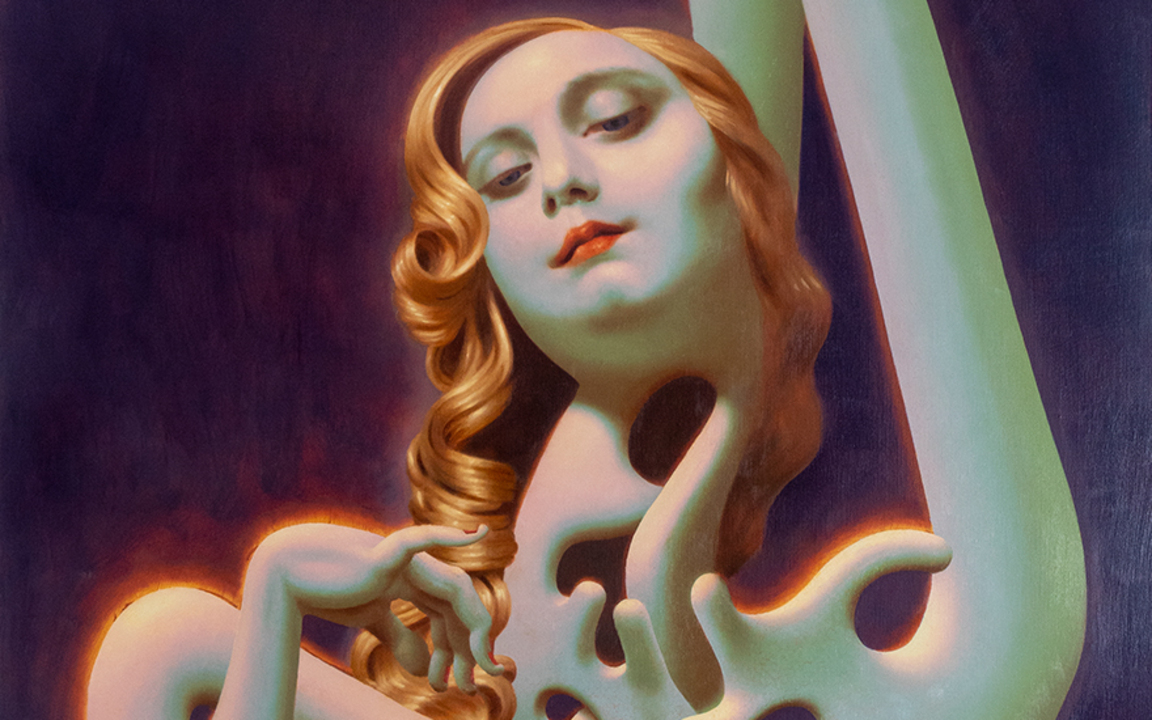This highly stylized, commercial art portrait features a woman with a dramatic and somewhat surreal appearance. She is centered in the image against a deep purple background. Her face is normal-looking but distinctly expressive, with her head tilted back slightly and her large, partially closed eyes gazing downward, giving the impression of both introspection and detachment. She wears orange lipstick, and her long, wavy hair is a vibrant orange-red, cascading down to the middle of her body.

Her neck is peculiarly open with hollow porcelain tubes emerging from it, swirling around in various directions. These tubes have an almost organic quality, one curving to the side of her head, another positioned behind her, and one bending as if symbolizing a knee. A particularly prominent one extends beside her head. The image includes a distorted, porcelain-like hand with fingers splayed and decorated with orange fingernail polish that matches her lipstick.

Her body has an abstract, disjointed structure, reminiscent of puzzle pieces, creating a fragmented and contorted appearance. The right side of the image shows an extended left arm with bony segments leading to a thin wrist and spread fingers. This adds to the surreal and slightly unsettling vibe of the artwork, making it a vivid, modern portrait with both sculptural and illustrative elements.